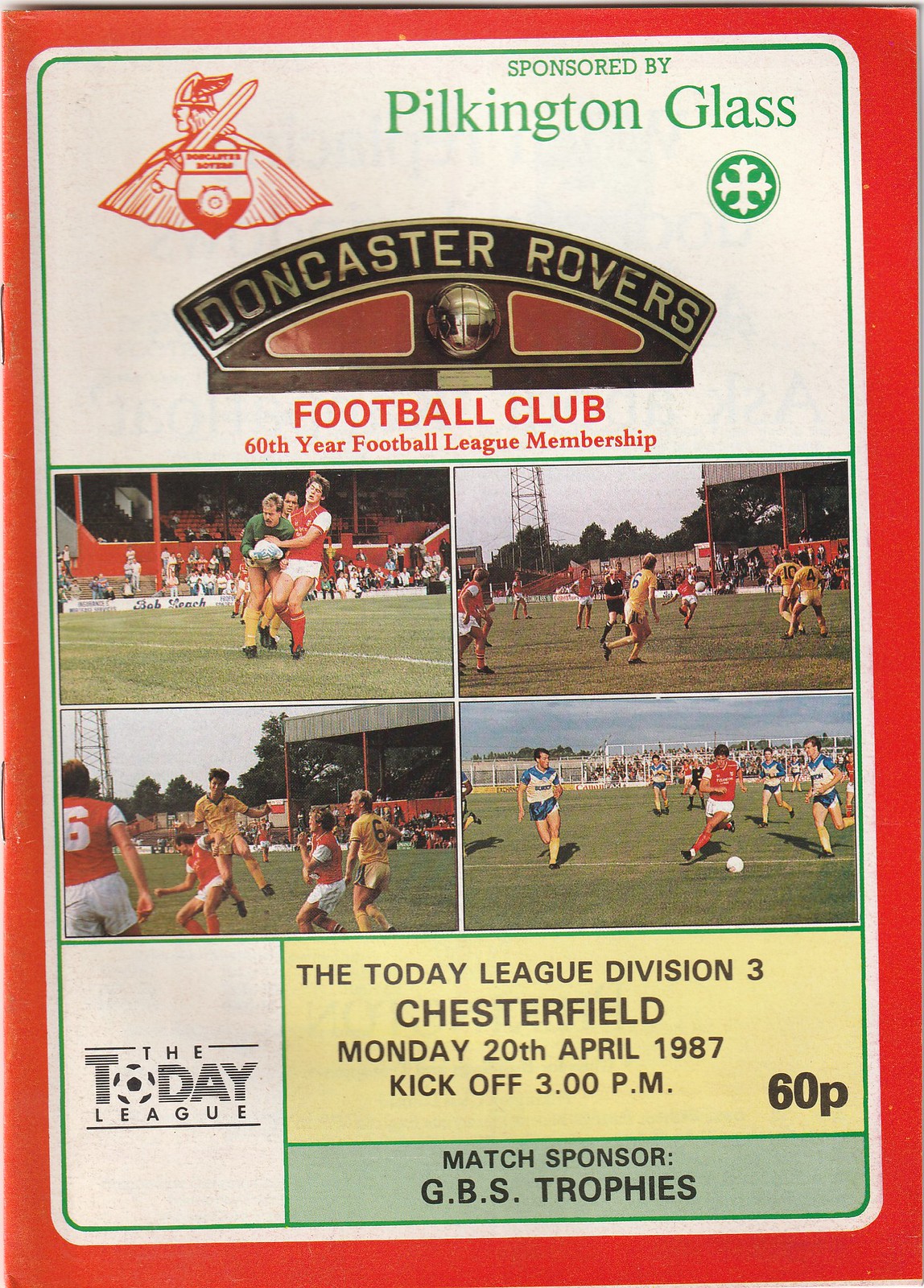This cover of a football program features a bold red border framing the content. At the top, there's a white section displaying the Doncaster Rovers logo, which depicts a Viking with a sword turned to the side. The text, "Sponsored by Pilkington Glass," is prominently written in green, accompanied by Pilkington Glass's green circle logo with a stylized white plus sign. The program celebrates the Doncaster Rovers Football Club's 60th year of football league membership, highlighted in a golden section with a soccer ball centerpiece resembling a trophy flanked by two red lines.

Beneath this title area, four photographs capture dynamic moments from recent soccer games, with the Rovers team easily identifiable by their red kits. The background in these images is a green playing field, and some shots include spectators in the bleachers.

Further down, in yellow text, it details the event specifics: "The Today League Division 3 Chesterfield, Monday the 20th of April 1987, kickoff 3pm, 60p." The design also features a playful touch where the "O" in "Today" is styled as a soccer ball. At the very bottom, in green, it notes that the match is sponsored by GBS Trophies. The overall layout is blocky yet colorful, combining reds, whites, greens, and yellows to create a vibrant and informative cover.